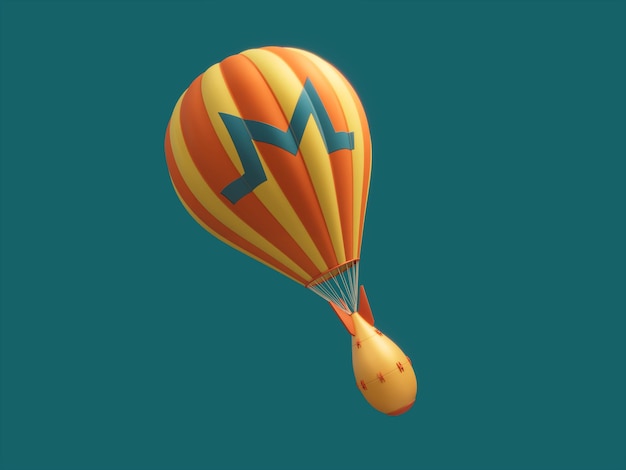This image appears to be a detailed illustration or 3D graphic of a whimsical balloon against a deep teal sky. The balloon resembles a hot air balloon with vertical stripes in shades of yellow and orange. At the top of the balloon is a large, stylized teal “M” with serifs at the bottom. Suspended by numerous strings, the lower part of the balloon deviates from traditional design, resembling an upside-down rocket or bomb in yellow with orange fins and possible star-like figures. The bottom section gives the impression of a playful child's toy designed to be thrown and watched as it descends, rather than an actual hot air balloon for human travel. The entire structure leans at a slight angle, as if blown sideways by the wind, adding to its fantastical and imaginative appearance.